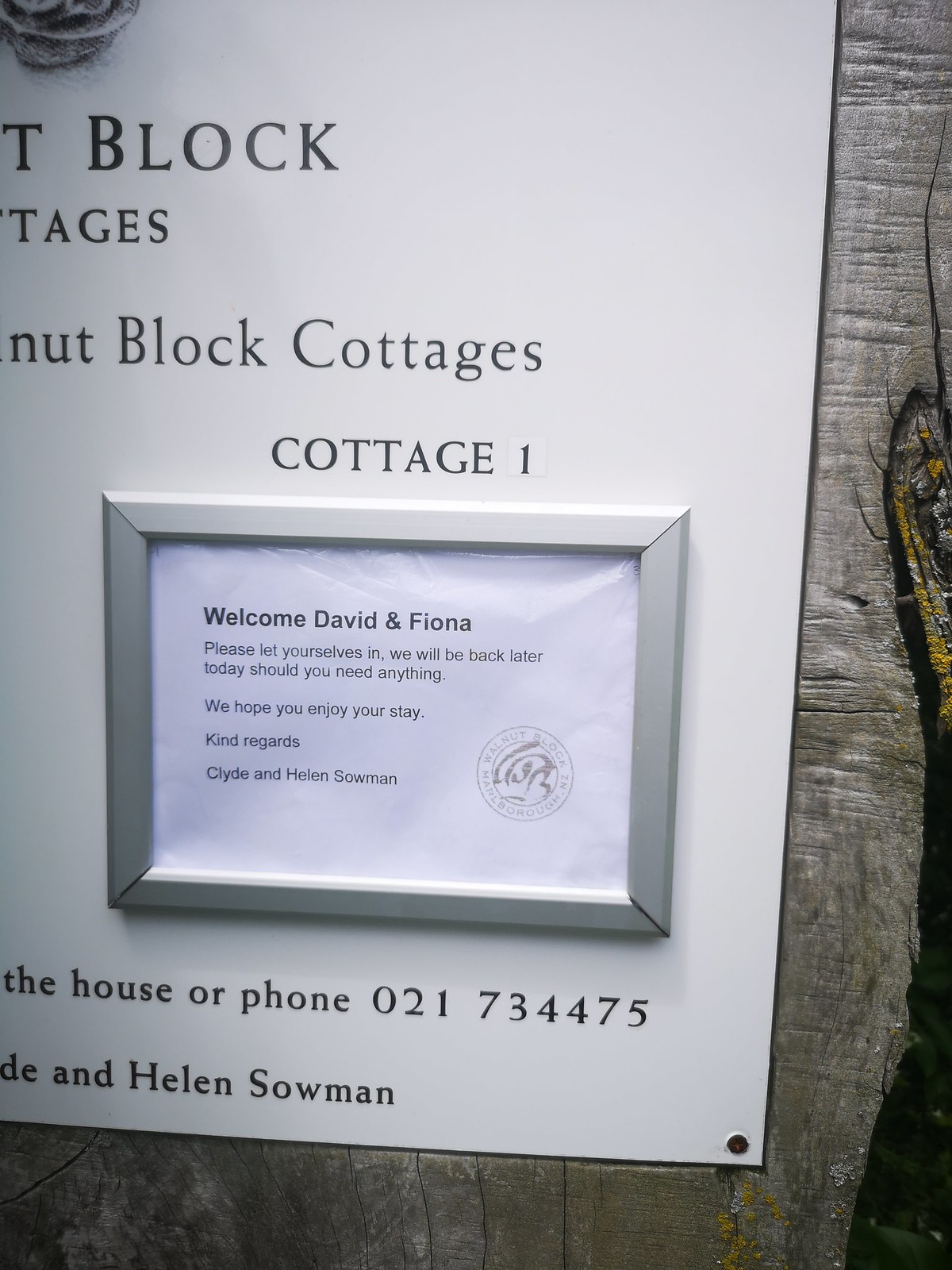This image, a color photograph in portrait orientation, captures a detailed scene at a Bed & Breakfast. The focal point is a sign or notice posted on a piece of white poster board placed within a silver wood frame. The board is affixed to a dark gray wood grain paneling wall. 

The note, centered within the frame, extends a warm welcome to guests David and Fiona. The text reads: "Welcome David and Fiona. Please let yourselves in. We will be back later today should you need anything. We hope you enjoy your stay. Kind regards, Clyde and Helen Snowman." The identical spelling of their surname is clarified as "Snowman." Below this text, the note specifies that the guests are to stay in Cottage Number 1, within a block of cottages. Further down, contact information is provided: "The house or phone: 021-734-475."

Partially cut off on the left side, the sign’s layout includes a logo in the bottom right corner of the framed paper, described as circular and silver, although its details are unclear. It represents a slice of careful hospitality, rendered in a realism style capturing the practical and inviting ambiance of the Bed & Breakfast.